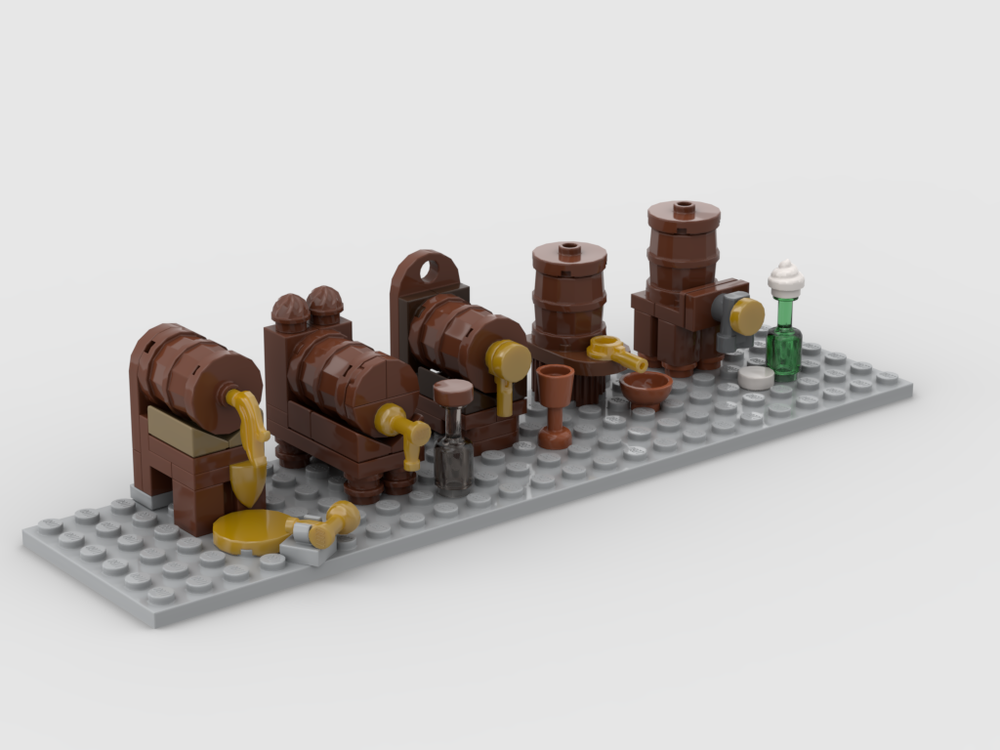The image showcases a detailed Lego set representing a brewery scene. The entire setup rests on a grey base plate with a plain white background, ensuring all attention is on the intricate arrangement of barrels and accessories. 

Five brown kegs are prominently featured: three are positioned horizontally towards the left while two stand upright on the right. Each keg shows different details:
1. The first horizontal keg is depicted with yellow liquid spilling out, forming a puddle below.
2. The second horizontal keg, fitted with a side tap, remains closed.
3. The third horizontal keg also has a closed side tap.
   
Between the second and third kegs is a green bottle, and beside the third keg is a mug, suggesting vessels used to collect the liquid. 

On the right side:
1. The first upright keg features an attached tap leading to an empty bowl, indicating it can dispense liquid.
2. The second upright keg, positioned at the far right, is closed and has a glass bottle placed in front of it.

The primary colors in this scene are the brown of the wooden kegs and the grey base plate, contributing to the realistic aesthetic of this miniature brewery setup.